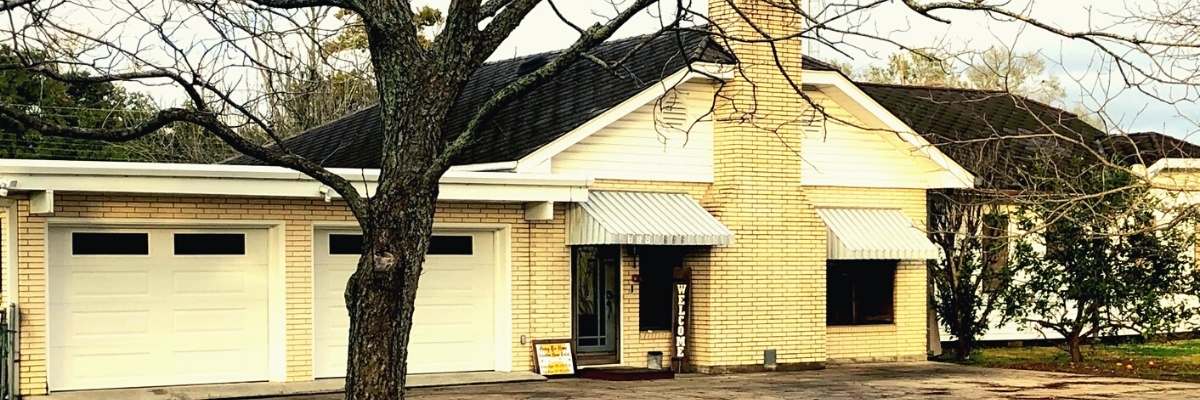The image showcases a single-story, ranch-style house with a yellowish-brick exterior, situated in a suburban neighborhood. Prominently featured is a large tree in the front yard, without leaves, indicating wintertime. The house has a two-car garage to the left, each door adorned with two horizontal rectangular windows at the top. Central to the facade is a tall, blonde brick fireplace chimney, flanked by windows with blue and white striped awnings. The front door, which has a gray trim, is under a yellow awning and features a large "Welcome" sign, suggesting it may be used as a business despite its residential appearance. In the vicinity of the welcome sign, there is another small, rectangular sign with yellow and white lettering, hinting at commercial use. Patchy grass and a large concrete slab are visible in the front yard, along with some dark green foliage. To the right of the house, a similarly colored neighboring house is partially obscured by trees and bushes.